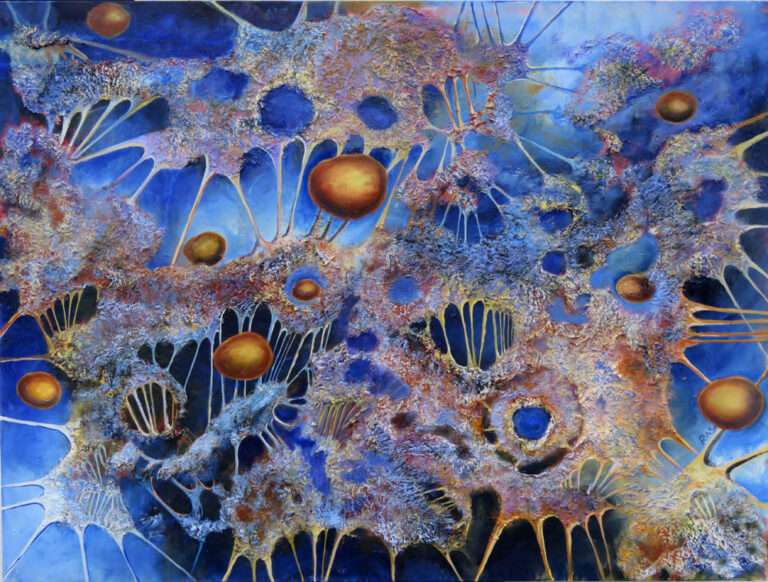The image is a detailed biological artwork, featuring a vibrant blue background with varying shades. Against this backdrop, a complex web-like structure extends across the canvas, reminiscent of either neural networks or bacterial colonies. The webbing is composed of yellow and orange tendrils that branch out, interconnecting different parts of the network. Scattered throughout the tendrils are round, sphere-like forms that are dark orange-brown at the edges, transitioning to a lighter yellow towards the centers. These spheres punctuate the structure, with some placed in the middle of the webbed blobs, enhancing the neural or microbial theme. Additionally, there are hollowed-out sections within the tendrils, allowing the blue background to peek through, adding depth and texture to the piece.